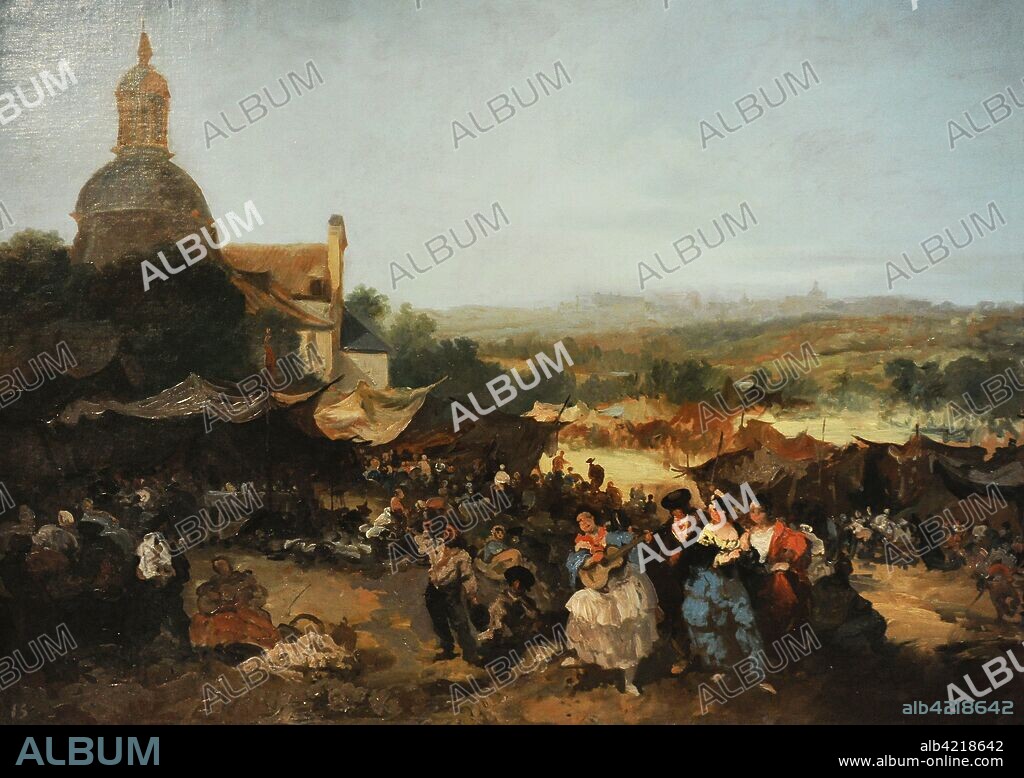The image depicts a vibrant, hand-drawn painting of a festive outdoor gathering, likely set during a fiesta or festival. Central to the scene is a woman adorned in a frilly dress, passionately playing a small guitar, surrounded by a mix of men and women either listening or interacting with her. The setting features a tent on the left, additional tents on the right, and a distant building, framed by trees and a fog-enshrouded town in the background. The landscape includes little hills and what might be undeveloped farmland, hinting at a location in Spain or Mexico. However, the painting is marred by numerous watermarks of the word "ALBUM" in varying styles, with some words outlined and others rendered in full white, detracting from the overall viewing experience. At the bottom, the word "ALBUM" appears again, alongside the URL "albumonline.com" in the bottom right corner, providing contact information and potentially an ID number for licensing or purchase.